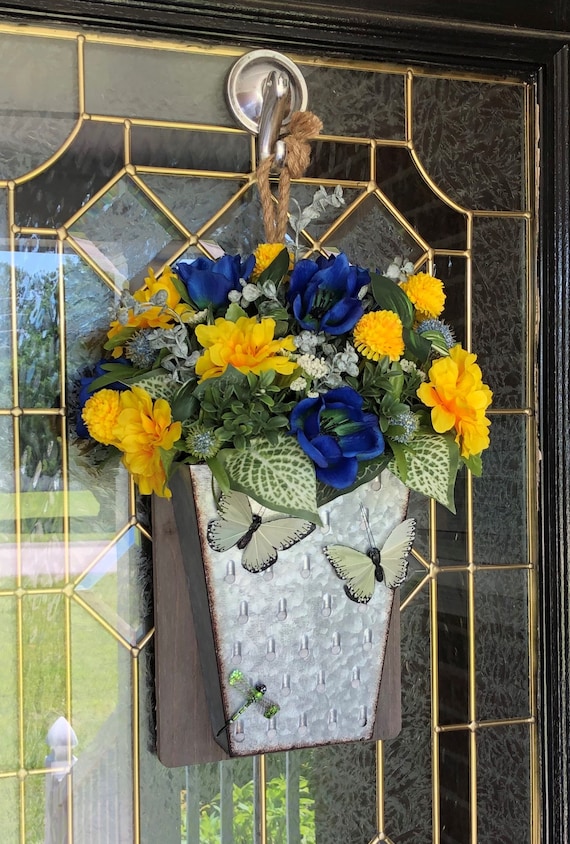This is a detailed photograph of a front door to a house that features an exquisite blend of etched and clear glass framed in black wood with gold trim around the panes. The centerpiece of the image is a decorative door hanger, secured by a silver nickel hook and suspended by a brown rope. The hanger consists of a silver-gray metal basket attached to a brown wooden base, overflowing with a vibrant array of flowers in royal blue, bright yellow, and white, accompanied by lush green and speckled green-and-white leaves. Adorning the basket are two white butterflies positioned near the top left and right, and a green dragonfly situated in the bottom left corner. The clear and etched glass offers a serene backdrop, subtly reflecting the porch, green lawn, and street beyond, adding depth and context to the scene.